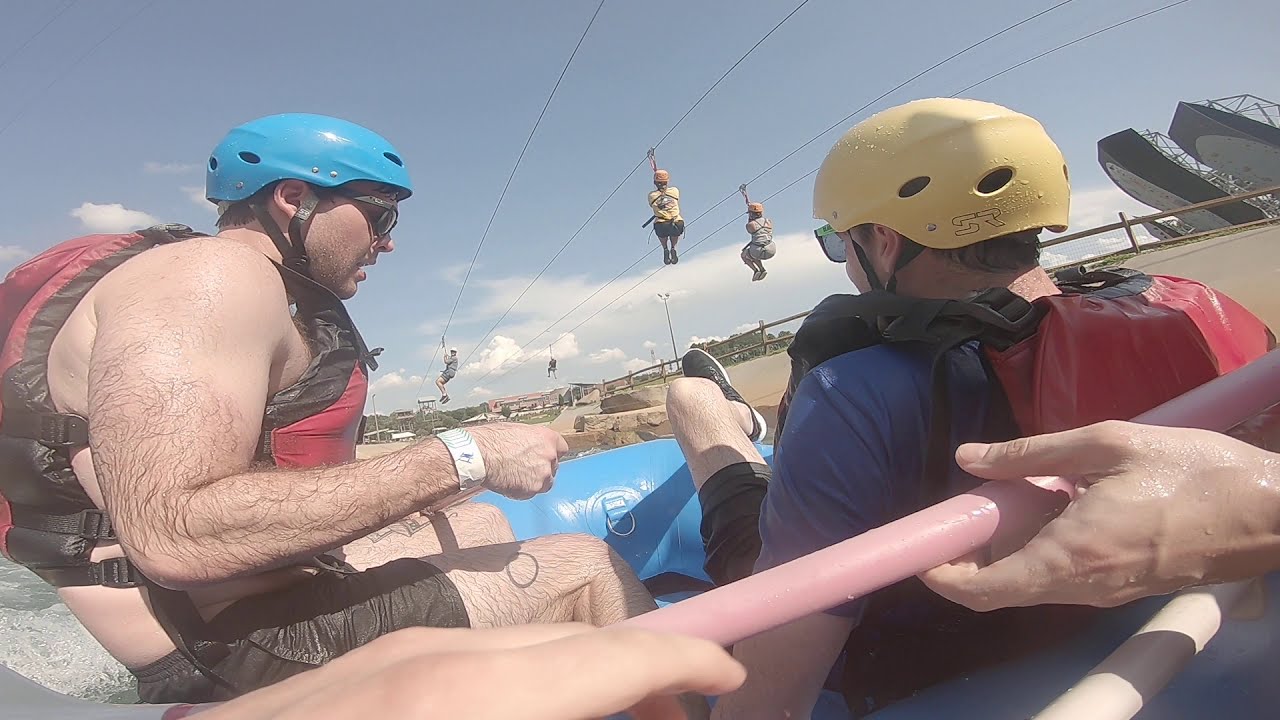In the sunny and hot early afternoon, an outdoor recreational area bustling with activity is depicted. Central to the image are two men riding an inflatable blue raft on a serene green river. The man on the left is dressed in a blue helmet and a red life jacket, while the man on the right sports a yellow helmet and a matching red life jacket. Above them, four individuals clad in casual attire—t-shirts, shorts, and helmets of various colors—are zip lining along cables, gliding through the blue sky dotted with white clouds. In the background, a distant bridge, multiple buildings, and trees complete the lively scene, further accentuating the vibrancy and diversity of the activities taking place.